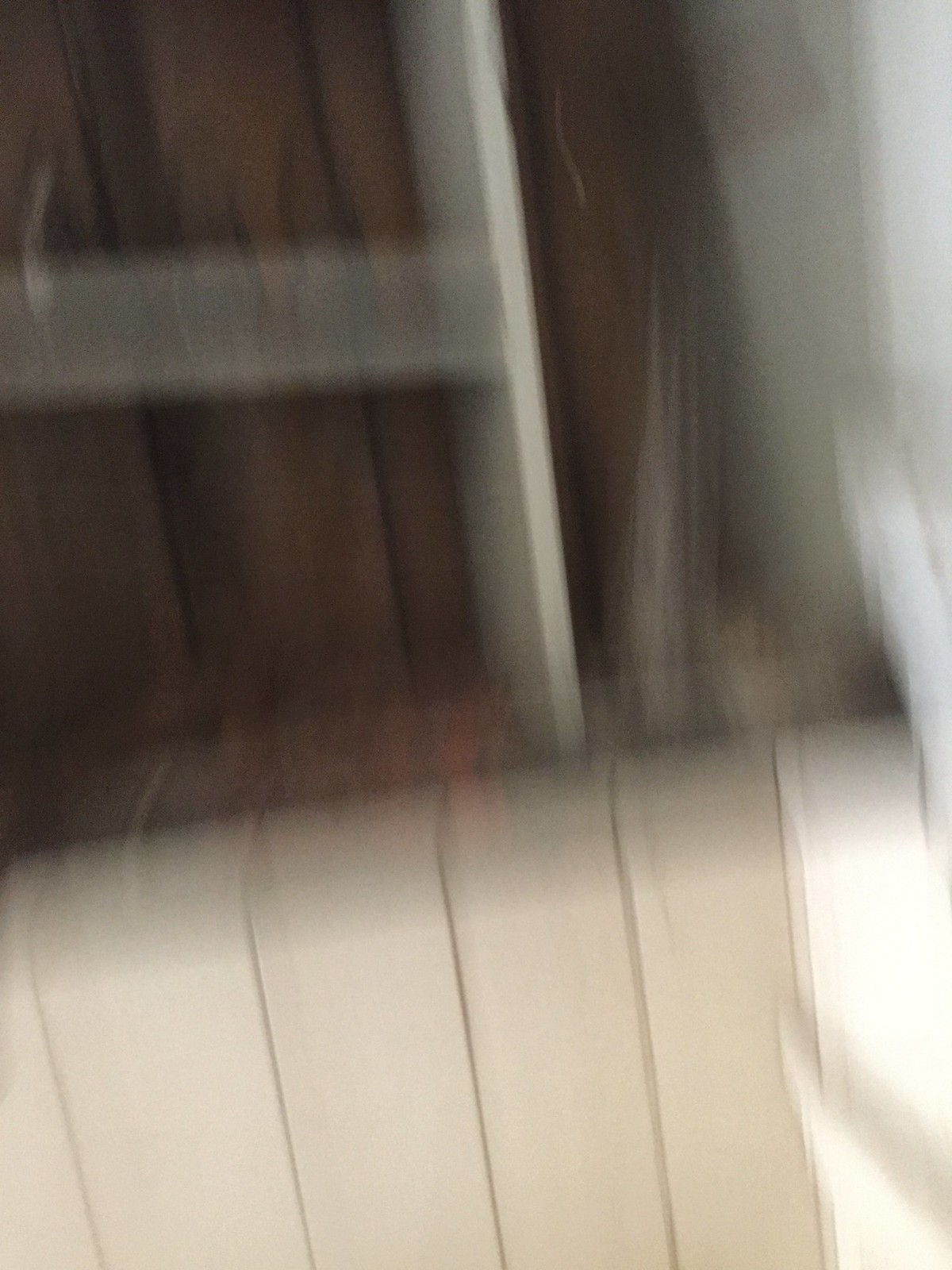This is a blurry photograph capturing the corner of a room. The primary focus is on a wall with vertical dark cream-colored siding. Against the wall, halfway up, there is a mounted unit that appears to be a combination of a bookshelf and a cupboard. The bookshelf has a vertical storage space on the right and a shelf on the left, with the right section seemingly having an open door. Additional details include an impression of a small, basic white shelf that rests on a ledge, which is defined by vertical light tan siding. Below this ledge, there are beige, vinyl-like straps reminiscent of a pool chair. The overall image is indistinct, with motion lines adding to the blur, making it challenging to discern further specifics about the room's function or contents.